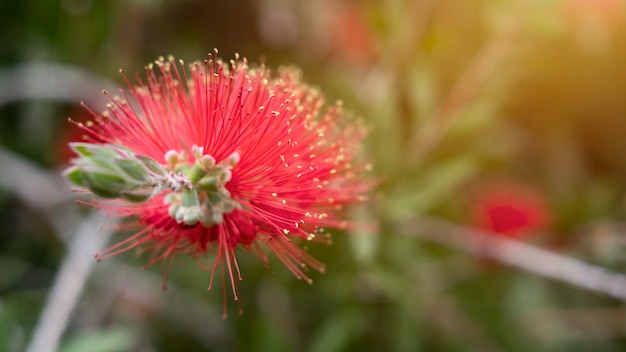The photograph features a unique and striking red flower occupying the left half of a rectangular image, which is wider than it is tall. The flower's structure deviates from typical floral forms, consisting of hundreds of thin, hair-like strands or straws radiating outward in all directions, creating a spherical shape. These strands are predominantly red or hot pink, each tipped with a tiny yellow dot, giving the impression of a red ball of fur sprinkled with minute yellow points. The central part of the flower contains clusters of green, oval-shaped buds or pods, suggesting that more of these hair-like strands might emerge from them. Around the flower's base, there are notably fewer and shorter strands, creating a fan-like appearance with a denser top and sparser bottom.

In the background, which is quite blurry, there is an indistinct, vegetative landscape. This backdrop includes patches of green foliage, elongated leaves, and additional red flowers of the same kind as the main subject, though they appear distant and out of focus. The right side of the image is characterized by brighter colors but remains unclear, with hints of stems or possibly branches looping around, adding to the complexity and depth of the scene. The overall effect is a vibrant, detailed portrayal of this extraordinary flower amidst a soft, verdant background.